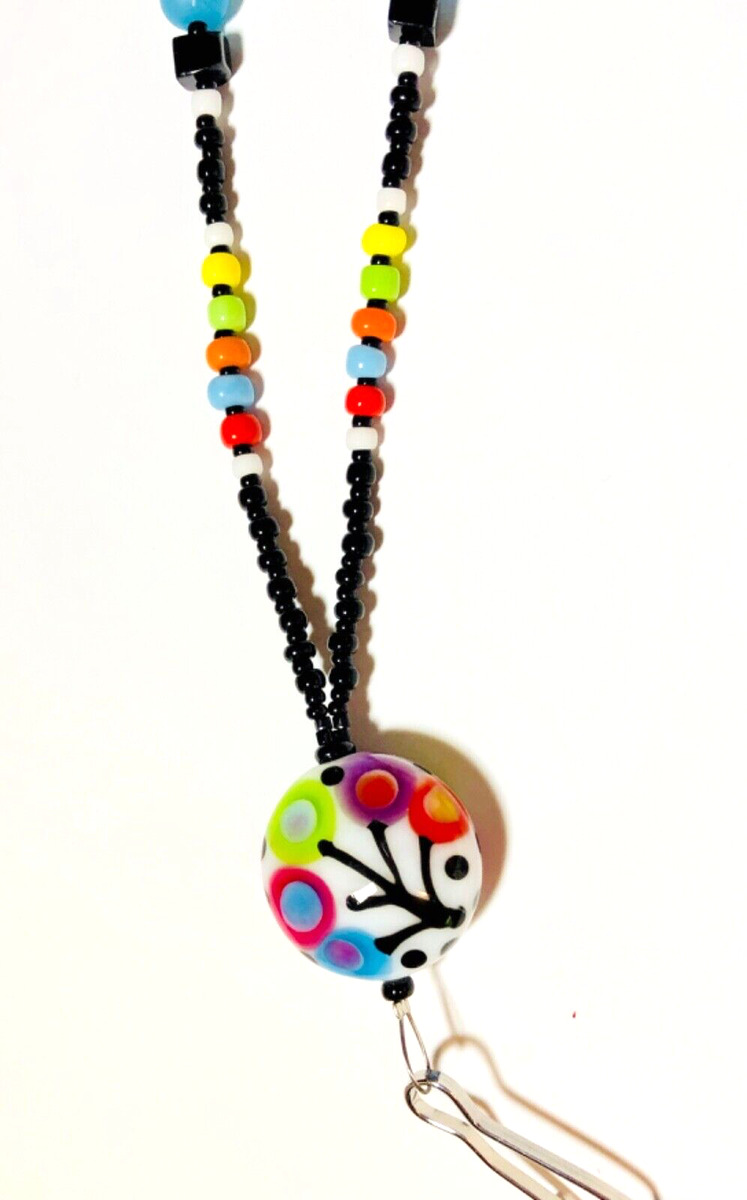This image showcases a close-cropped photo of a beaded lanyard set against a cream-colored background, taken from above with indoor lighting casting a shadow. The lanyard is composed of two strands adorned with beads. Each strand features alternating patterns of black and white beads, followed by a sequence of black beads interspersed with colorful ones in various shades such as yellow, green, orange, blue, red, and more, culminating in two black cubes at the top.

At the center of the lanyard is a striking, flat circular pendant. This pendant is primarily white and decorated with a black tree-like pattern featuring five branches. Each branch ends in a colorful circle with an inner dot, showcasing various color combinations like blue-purple, red-blue, green-white, purple-red, and red-yellow. This central pendant attaches to the bead strands and further connects to a smaller black bead and a metallic, carabiner-like key hook at the bottom, suggesting that this item functions as a lanyard.